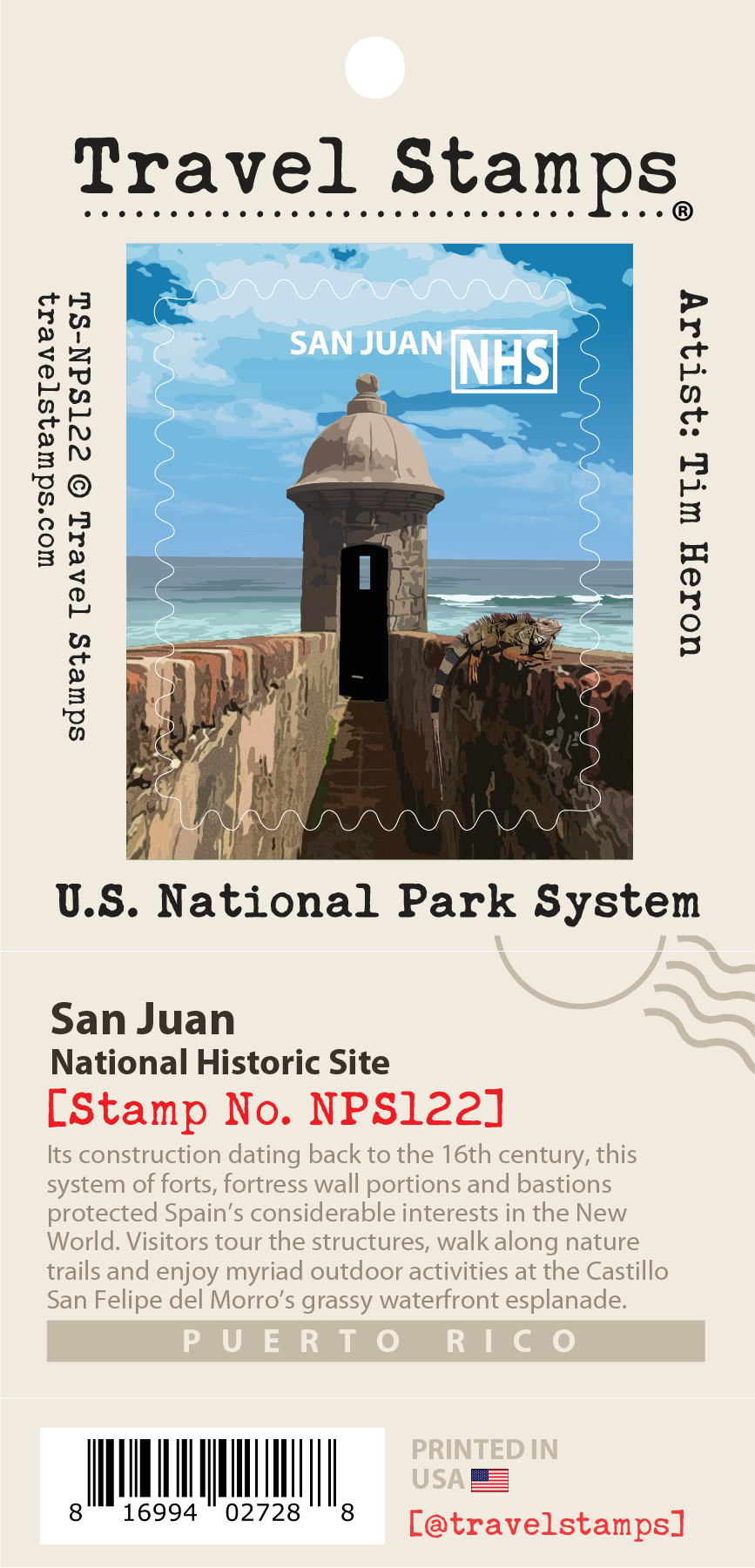This image depicts a cream-colored travel stamp for Puerto Rico, specifically the San Juan National Historic Site. Set against a beige background, the rectangular stamp features a circular hole at the top and bold black letters that read "Travel Stamps," with a line of dots beneath. Below this, a small, detailed picture showcases an old, brown tower with a small window in the middle, capped at the top, and set against a blue sky with large white clouds. This tower, part of the Castillo San Felipe del Morro, stands by the ocean and hints at a larger fortress system built by Spain in the 16th century to protect their New World interests. The tower is connected by a concrete-looking walkway flanked by two walls, with a small brown lizard visible on the right wall. 

The image on the stamp has "San Juan NHS" written on it, indicating the site’s affiliation with the U.S. National Park Service. To the right of the picture, the artist's name, Tim Heron, is written vertically. Beneath the picture, it says "U.S. National Park System" and "San Juan National Historic Site," followed by the stamp number "NPS 122" in red lettering. At the bottom left corner, a barcode is present, along with the note that it was printed in the USA.